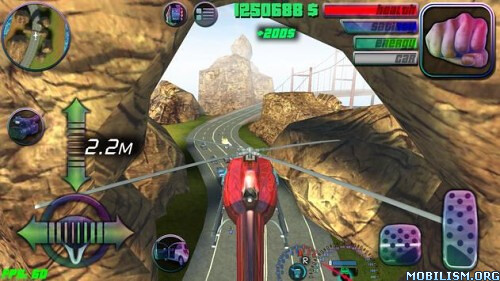In this detailed video game screenshot from a mobile game, the view is uniquely set in landscape mode, offering an immersive experience uncommon for most mobile games. The player's vehicle, a red helicopter, is prominently displayed against a backdrop that hints at a lower resolution and budget-friendly graphics. At the top of the screen, the current in-game currency amounts to an impressive $1,250,688.

The user interface is rich with information: the top right corner features multiple bars representing health, mana, energy, and potentially power, the latter indicated by a fist icon. The top left corner houses a mini-map, aiding navigation. The bottom left corner showcases a steering wheel flanked by directional arrows for steering left and right, with green arrows above these for ascending and descending, denoted further by a "2.2m" label.

In the bottom right, the display resembles an automobile's control setup with both gas and brake pedals, accompanied by a speedometer to the left. Additional, albeit indistinct, icons populate the screen, adding layers of functionality. The red helicopter is seen flying over a highway, which is scenically surrounded by mountains and features a striking natural arch of rocks overhead. The overall setting suggests a diverse and visually engaging in-game environment.